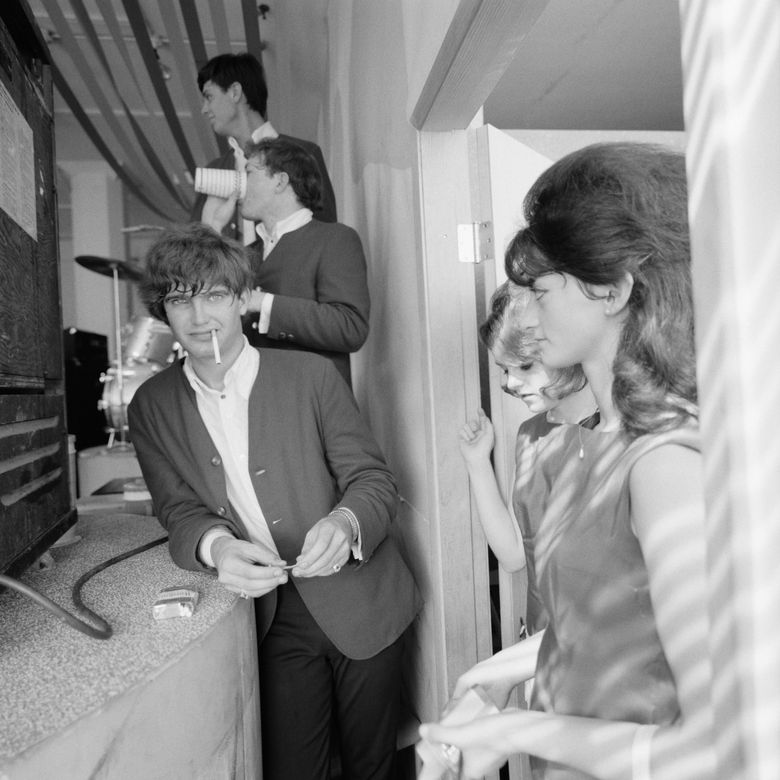This black-and-white photograph appears to be from the 1950s or early 1960s and features three men and two women. The scene is set behind a stage, with a visible drum set positioned on the far left. Positioned in a staggered formation, the three men all wear collarless jackets with white shirts. The man in the foreground, leaning against what seems to be a shelf, has a cigarette dangling from his mouth and a matchbook in hand, gazing directly at the camera with a slight smirk. Behind him, a second man is captured mid-drink from a white paper cup. The third man stands at the top of the steps, looking thoughtfully into the distance. To the right, two women are seen standing in a doorway. The woman closest to the camera sports dark, bouffant-style hair and a small pearl necklace, dressed in what looks like a gray dress. Behind her, a blonde woman also has volumized hair and appears to be looking down, adorned with a similar pearl necklace. The overall composition and fashion details strongly evoke the mid-20th century ambiance.